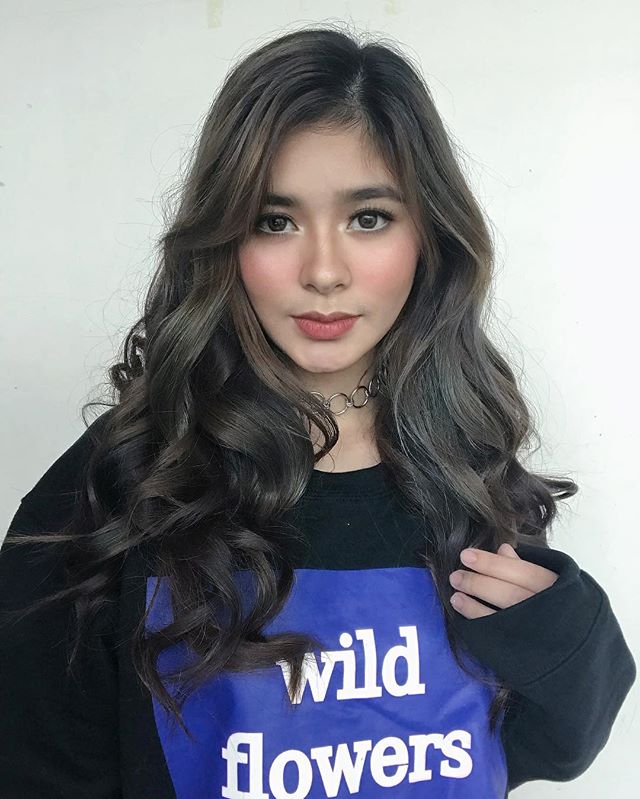In the image, a young woman in her early 20s stands against a flat, grey background. Her long, wavy brown hair flows around her face, becoming even wavier towards the bottom. She has bushy brown eyebrows and brown eyes adorned with light pink makeup that adds a subtle blush to her cheeks. Her full lips are painted red. She is wearing a heavy, black sweater with a blue square on the front that reads "WILDFLOWERS" in white, uppercase letters. Around her neck is a silver chain necklace made of circular links. One of her hands, with clear, unpainted nails, is raised to touch the bottom of her hair. In the background, there are two small pieces of yellow tape visible, positioned above her head towards the center and right. Despite the minimalistic setting, the details of her appearance capture a sense of depth and personality.